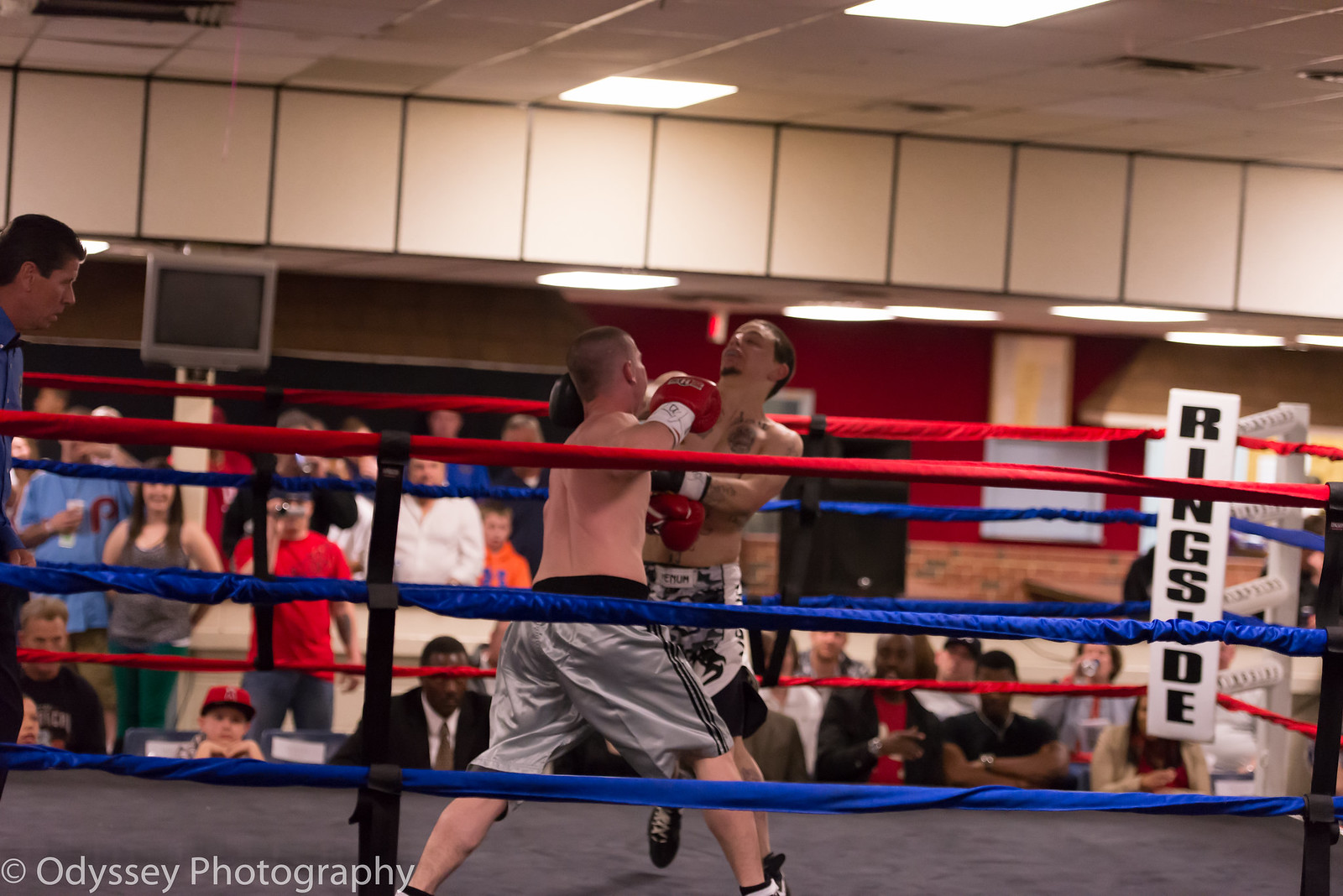The photograph captures an intense moment inside a small boxing ring during an official match. Two Caucasian male boxers are at the center of the action; one boxer, wearing red gloves and grey shorts, appears to have just landed a punch on the other boxer, who is donning black gloves and black and white shorts. The impact is evident as the latter's head is thrown backward, possibly signaling he is about to fall. To the left, the referee, dressed in a blue shirt and black pants, is partially visible, ensuring the bout's regulations are followed. 

The boxing ring is enclosed by three ropes wrapped in cloth, with the top rope being red and the middle and bottom ropes being blue. A white sign with black lettering reading "RINGSIDE" is positioned in one corner of the ring. Surrounding the ring, an audience of about a dozen or more spectators is energetically watching the fight, with some capturing the action on video. Among the crowd, a white male wearing a red shirt and blue jeans is conspicuously recording the match. The bottom left corner of the photo bears a copyright symbol with the text "Odyssey Photography," authenticating the image. This snapshot vividly portrays the intensity and dynamics of a competitive boxing match.